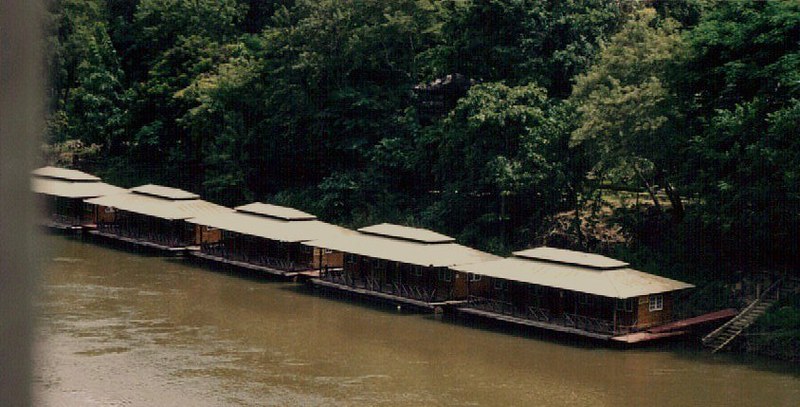This photograph, set along a riverbank in a dense jungle, captures a series of five identical wooden hut houses, resembling stationary houseboats. These rectangular structures are crafted from dark brown wood with light tan, gazebo-like roofs featuring vents at the top. Each house has a white-trimmed window arrangement, with four windows in the front and additional windows on the sides. They boast sizable porches and interconnected decks, offering views over the dark, muddy-brown water, likely tinted by natural elements. A staircase on the right leads down to the river, with a walkway connecting the houses. The background is filled with dense greenery, thick foliage of green-leaf trees that frame the scene, adding to the serene and rustic charm of the location. On the left edge of the image, there's a blurred white object, contributing to the overall mystique of this quaint riverside setting.